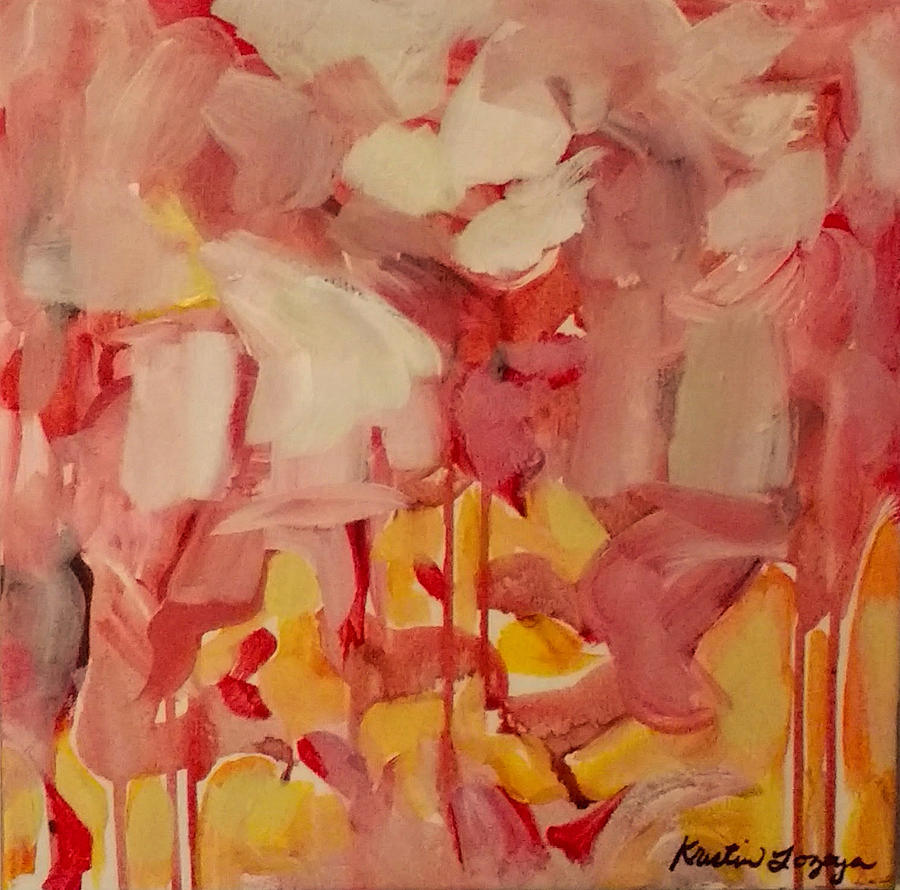This image depicts an abstract floral painting by the artist Christine Lonzoya. The top half of the painting is dominated by an array of pinks, from light pastel shades to dark magenta, and brick red, forming abstract flower shapes with wide and thin brushstrokes. The bottom half features red stems and scattered leaves against a luminous background of mixed dark and light yellows, evoking the impression of a vibrant field of flowers. The painting also includes the artist's signature, "Kristen LaZoya," subtly placed in black in the lower right corner, confirming the artist's identity. The overall composition creates a dynamic and colorful representation of an abstract floral landscape.